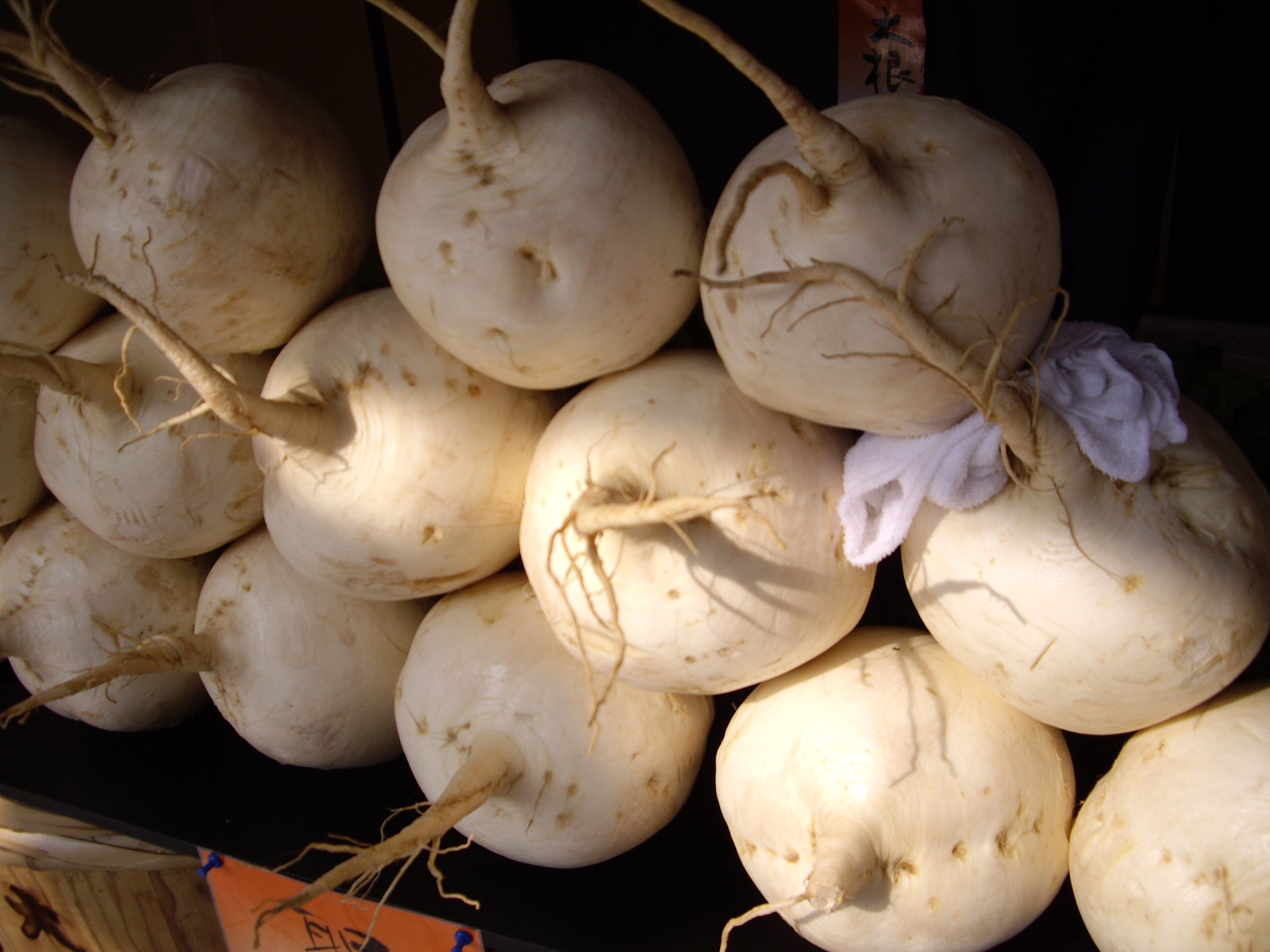The image depicts approximately 14 white, robust, root-tipped vegetables that appear to be turnips or members of the squash family, arranged on a dark, most likely black, shelf. The vegetables are stacked in three rows with some sitting on top of each other, and there's a literal white cloth tucked between two of them in the upper right corner. The background includes a wooden area below the shelf with an orange sign pinned to it using navy blue thumbtacks. The scene is bathed in streaks of sunlight, suggesting that it is likely morning. Below the shelf, there is potentially a tin garbage can, though this detail is less clear.